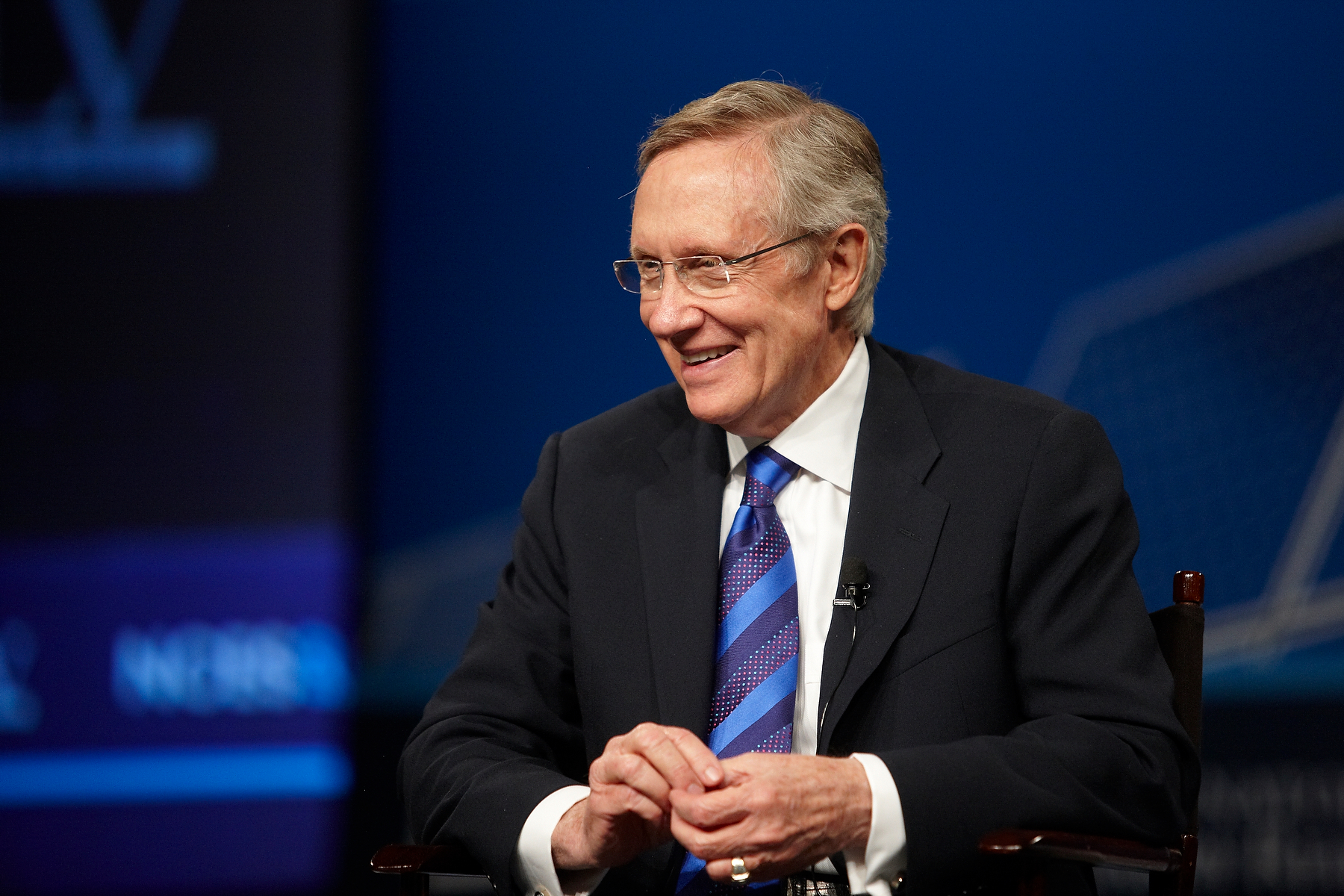A white-haired, bespectacled man sits comfortably in a simple chair, laughing and looking to his left. His thin-framed glasses, rectangular in shape, rest lightly on his face. He is attired in a sophisticated suit, featuring a black jacket, a crisp white collared undershirt, and a multicolored striped blue tie. His hands are clasped in front of him, fidgeting slightly, with a noticeable ring adornment on his pinky finger. The backdrop consists of multiple television screens, some of which emit a blue hue, adding an electronic ambiance to the setting.